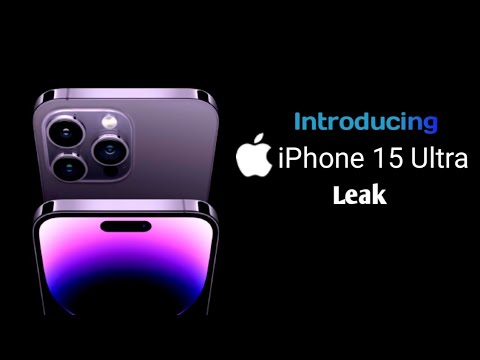A meticulously crafted, yet unofficial, promotional image captures the anticipated excitement around the rumored iPhone 15 Ultra. The composition cleverly mimics the sleek and sophisticated style typical of Apple's advertisements, with the phrase "Introducing iPhone 15 Ultra" prominently displayed at the top in a gradient of blue tones that darken towards the edges, accompanied by the iconic Apple logo. Below, the word "leak" suggests this is an unreleased, speculative sneak peek.

In the image, two iPhones are artistically stacked against a stark black background. The phone positioned lower and to the left showcases the front, revealing a vibrant, graded screen with precise metal framing. The device above and behind highlights the back, featuring a light-gray finish and the recognizable tri-camera array, complete with minute reflections on the polished metal surface. The overall aesthetic captures the essence of an Apple ad, designed to intrigue and captivate, even though it subtly discloses its unofficial nature through the telltale "leak" designation. This mockup serves as a tantalizing glimpse into the possible future of iPhone design, crafted to attract attention and stimulate conversation among tech enthusiasts.